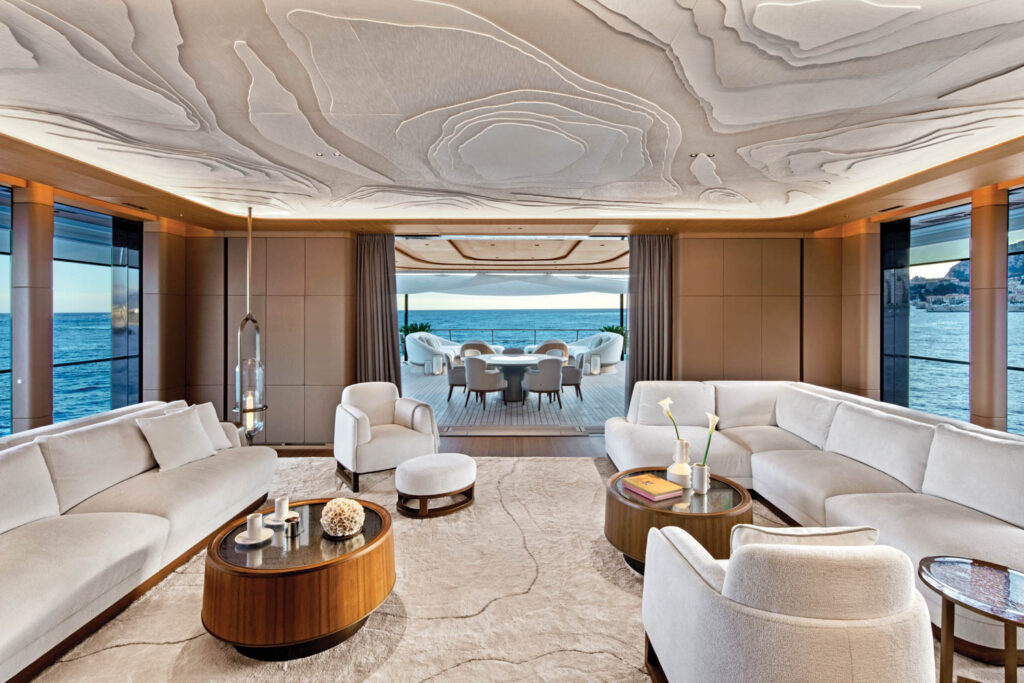The image depicts a luxurious, beautifully set room aboard a boat, surrounded by the vast, serene ocean. In the room, there are two white sofas—one on the left and a larger one on the right—both adorned with matching white cushions. A white chair accompanied by a white footstool with brown legs is positioned in the front. On the left side of the room, a table with a reflective surface and a brown body holds two cups, each placed on a saucer, along with a candle holder. The room also features round wooden coffee tables, adding to its high-class ambiance. The eye-catching ceiling has a unique design composed of layered shapes in beige tones. Visible through the windows is the picturesque sea, with a glimpse of land in the top right corner of the picture, further accentuating the room's opulent and tranquil setting.